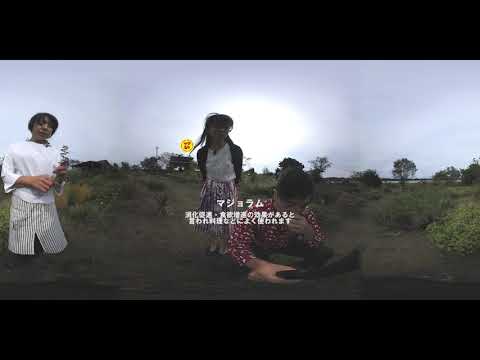This horizontally aligned rectangular image, bordered by thick black bands at the top and bottom, showcases three individuals standing outdoors on a dirt and grass area with scattered trees under a cloudy sky with the sun peeking through. All three appear to be of Asian descent. On the left, a woman with black hair, possibly pulled back in a ponytail, is dressed in a white blouse and a finely striped white skirt. She is holding an item (potentially a plant or flower) in her hands and faces the camera. In the center is another woman with glasses, longer dark hair, a white blouse, and a longer skirt. In front of her, slightly blurred, crouching down, is a figure (gender unclear) with black hair and bangs, wearing a red and white shirt. This person seems to be holding something in their right hand and has one hand to their mouth. The scene is overlaid with white text in Chinese or Japanese characters, suggesting it might be a low-resolution still from a movie or a screenshot from a TV ad.